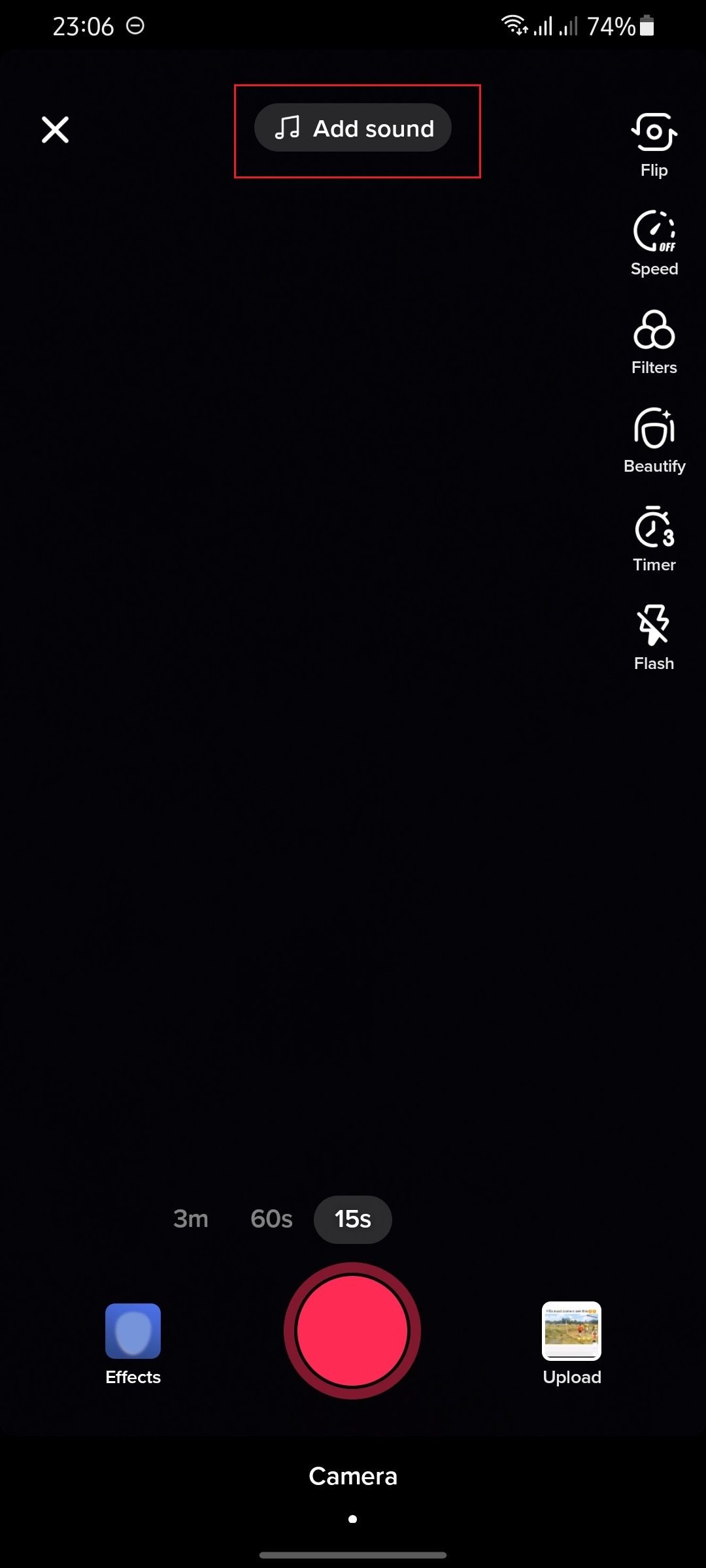The digital image appears to be a screenshot taken from a smartphone, displaying the interface of a camera application. The time is shown in military format as 23:06 and the battery level is at 74%. The interface includes various options, such as adding sound, flipping the camera, adjusting the speed, applying filters, using the beautify feature, setting a timer, and turning the flash on or off. Currently, the camera timer is set to 15 seconds, with additional options available for 60 seconds and three minutes. The main button to capture an image is a prominent large red circle, labeled "Camera" in white text above it. There is also a small white dot beneath this button, which likely indicates an upload status or connectivity rate.